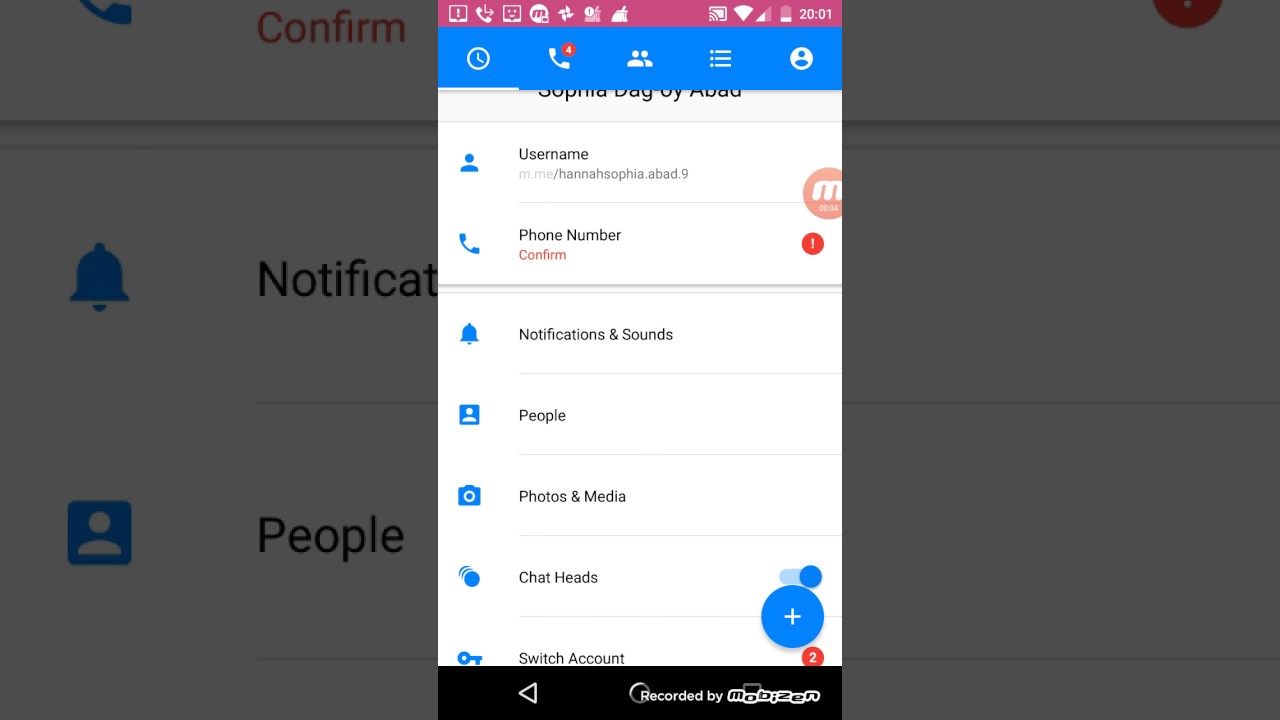The image features a predominantly purple background with some faint, printed text that reads "Confirm Notifications and People," accompanied by blue icons. The background appears slightly fuzzy. Overlaying the background, there is a page with a purple header displaying various icons. On this purple header, there is a blue box that includes a clock and phone icon with a small red circle containing a white number inside it. Additionally, there are icons illustrating people and lines with dots beside them, as well as a circular icon featuring a person.

Below this header, there is some black text that appears to be cut-off, partially revealing a username and phone number field, followed by a pink "Confirm" button. To the far right, there is a red circle with a white "M" inside it and a smaller red circle adjacent to it containing the number "1."

The page also lists various settings options such as "Notifications and Sounds," "People," "Photos and Media," "Chat Heads," and "Switch Account." To the right of these options, there is a prominent blue circle with a plus sign, accompanied by another blue circle above it and a shadowy blue shape beside it. Towards the bottom right corner, there is a red circle containing the number "2." The bottom of the image features a black bar with a left-facing arrow and the text "Recorded by Mobizen" in white.